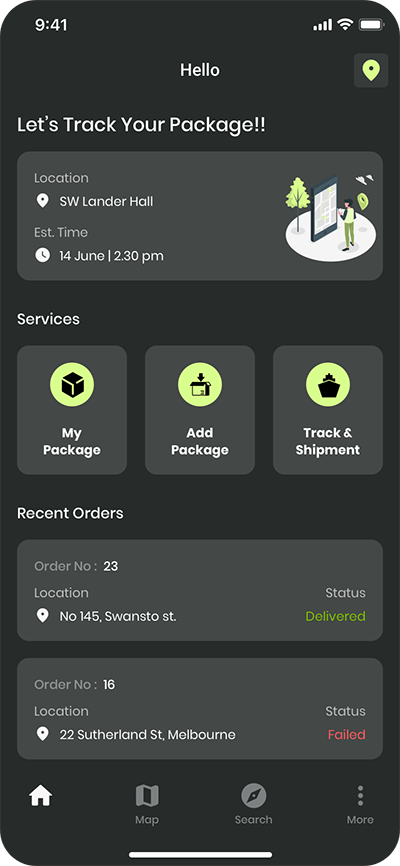This image is a screenshot of a package tracker app interface on a smartphone. The background is predominantly black, fitting within a vertical rectangle format. 

In the status bar at the top, the time "9:41" is displayed in white text on the top left corner. Adjacent to it on the right side, there are connectivity bars, followed by the Wi-Fi signal icon, and the battery indicator icon.

Beneath the status bar, in the center, the screen greets with "Hello" in white text accompanied by an upside-down teardrop directional icon to the right.

Further down, on the left side, the phrase "Let's track your package!" invites user interaction. Directly underneath, a charcoal black rectangle provides tracking details. The rectangle contains white text stating "Location: West Lander Hall," followed by an estimated delivery time, "14 June, 2:30 PM." To the right of this information, there's a small cartoon illustration of a man standing in front of a directional map in a park with a tree in the background.

Below this section, the word "Services" appears in white text. Beneath it, three smaller charcoal black boxes are aligned horizontally:
1. The first box shows a neon green circle with a small black box inside, labeled "My Package" in white text below.
2. The second box displays another neon green circle with a box inside, labeled "Add Package."
3. The third box features a similar neon green circle with a distinct box design inside, labeled "Track and Shipment."

Following this section, the screen shows "Recent Orders" in white text, followed by two rectangles displaying order details:
1. The first rectangle lists "Order Number: 23," "Location: 145 Aswanso Street," and "Status: Delivered."
2. The second rectangle provides details for "Order Number: 16," "Location: 22 Sutherland Street, Melbourne," with the status marked as "Failed."